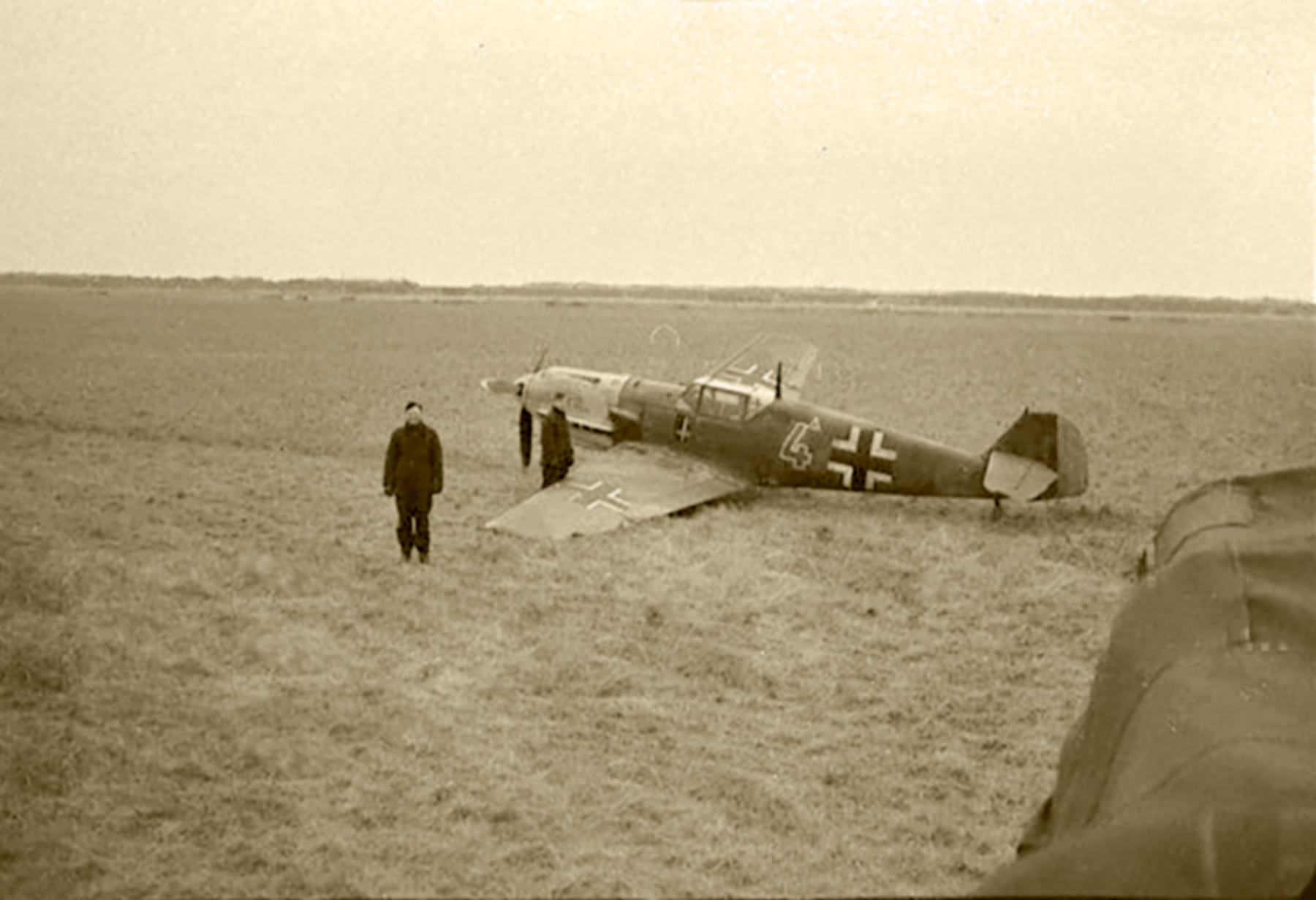This vintage photograph captures a World War II scene featuring a crashed German fighter plane, identified as a Messerschmitt. The aircraft is situated in a field and is leaning on its left wing. Despite the crash, the plane remains mostly intact. The single-engine fighter, with its distinct forward-mounted propeller, exhibits the German cross insignia prominently on the wings and tail. Notable details include the number "4" painted right behind the cockpit, with the engine sporting a lighter gray shade compared to the darker gray body of the plane. Two men stand to the left of the aircraft, one nearest to the wing and the other slightly forward and closer to the camera. The overall composition of the photograph, taken from an outdoor field under a monochromatic palette of black, white, and gray, emphasizes the historical and wartime context of the scene.